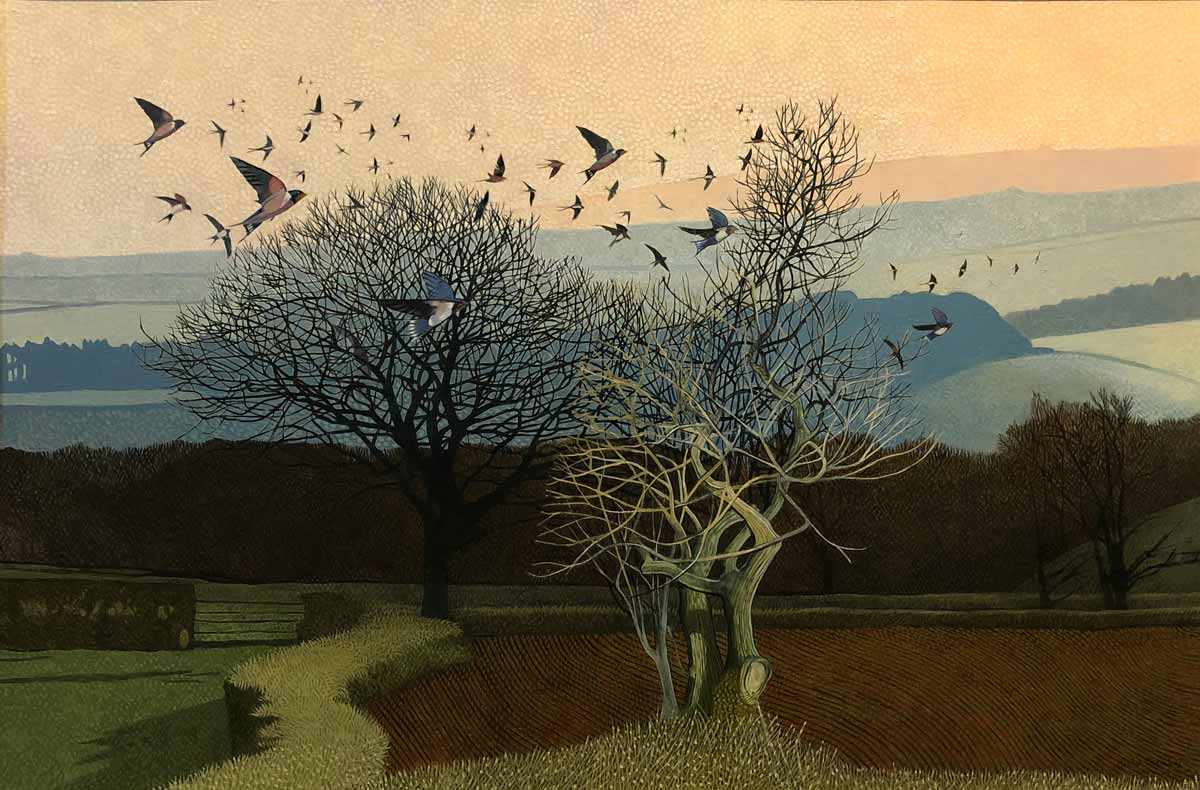The painting depicts a serene, muted outdoor natural scene showcasing a central cluster of bare trees whose branches transition from a white-ish hue to darker brown. A dense flock of around 30 birds, potentially sparrows given their red-tinted wings and white breasts, are depicted in flight, predominantly heading towards the right side of the composition. In the lower left corner, a low, cream-colored hedge blends seamlessly into the surrounding field areas, which exhibit a mix of fallow land and sparse greenery. In the background, rolling hills of blue and green tones ascend into a pink-hued sky, their silhouette stark against the horizon, while a distant river and some silhouetted mountains can be discerned. Several details, including a fence and a gate near the base of the trees, enrich the scene, with the subdued palette of pale pinks, blues, and earthy reddish-browns enhancing the painting's tranquil yet slightly somber atmosphere.